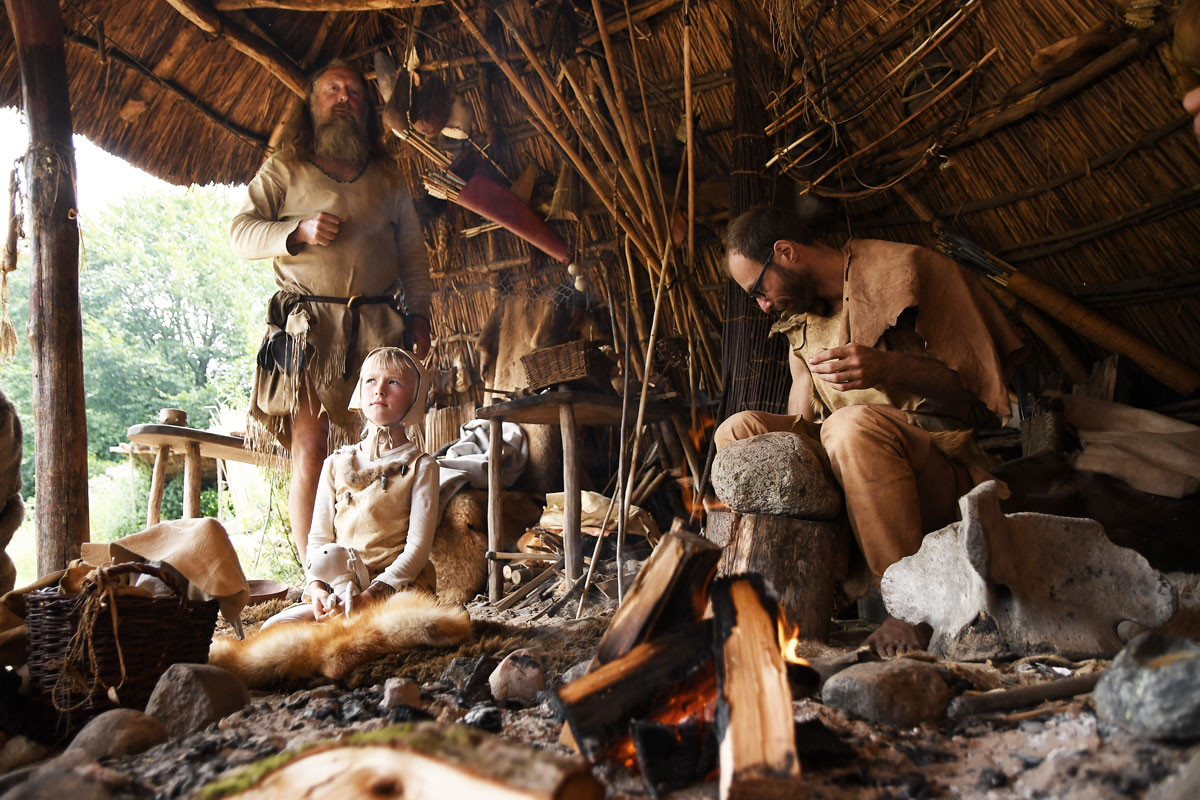In the photograph, there is a detailed depiction of a historical reenactment scene taking place inside a thatched hut. The structure is made of dark brown wood and grass, with a straw roof, creating an authentic setting that recalls ancient times. Situated under the hut, a rustic atmosphere is emphasized by the scattered sticks and the campfire’s orange embers glowing below large pieces of burning wood.

On the right side of the image, a man with short dark hair, a full beard and mustache, and dark-rimmed glasses is deeply engrossed in his woodworking craft. He is seated on a rock, leaning over a long horizontal piece of wood that he is carving, working against a stone. Dressed in a short-sleeve brown shirt or smock and khaki trousers, he gives the impression of a dedicated artisan reminiscent of early American settlers or Neanderthals.

To the left, a young girl with blonde hair and a traditional leather headdress sits on the ground, holding a carved white bunny rabbit toy in her lap. She wears a light yellow vest with white sleeves, fitting the historical attire. Standing behind her is an older man with a gray and white beard, donning a long cream-colored shirt with black and white string drapes, complementing the scene with his period-accurate clothing.

In the background, outdoor elements are visible through an opening on the far left side of the hut. Brightly foliaged trees and a wooden workbench reinforce the natural, rustic ambiance. The overall scene appears to be a demonstration, potentially showcasing life during the Neanderthal period or the era of early American pilgrims, with lifelike wooden figures and traditional activities bringing history to life.